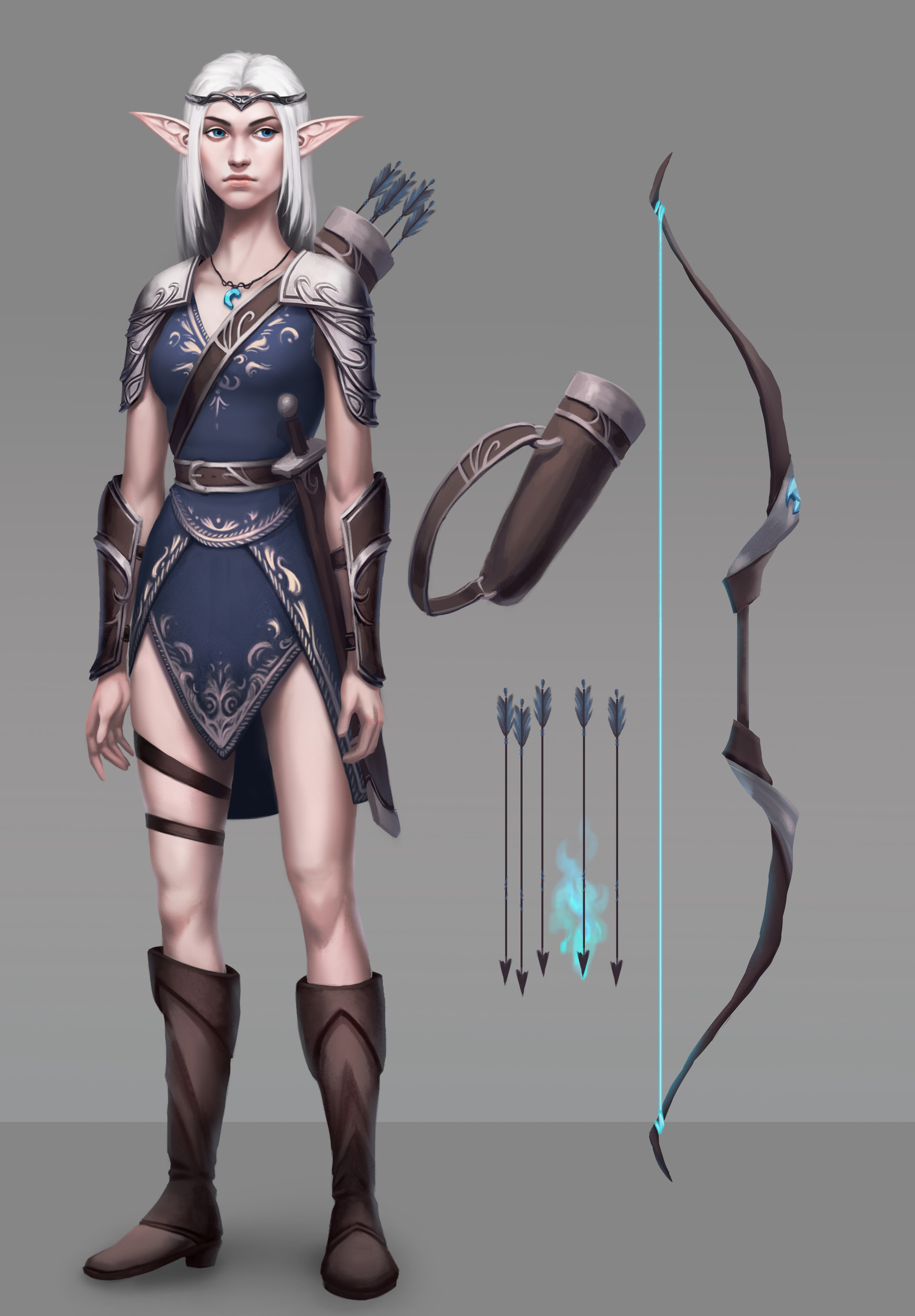The image depicts a female elf-like character, likely from a video game, positioned on the left side of a grey background. She has striking white hair and large, pointed ears. Clad in dark blue armor that resembles a dress, she also sports knee-high brown boots with heels, leather straps on her right leg, and leather armor on her forearms and shoulders. A quiver with several arrows, including a distinctive blue poison-tipped arrow, is fastened to her back. Holding a long black bow strung with a light turquoise string, she is accessorized with a necklace featuring a green, curved moon-shaped ornament. Her large blue eyes add to her otherworldly appearance, making her a quintessential archer character suitable for a video game or folklore setting.